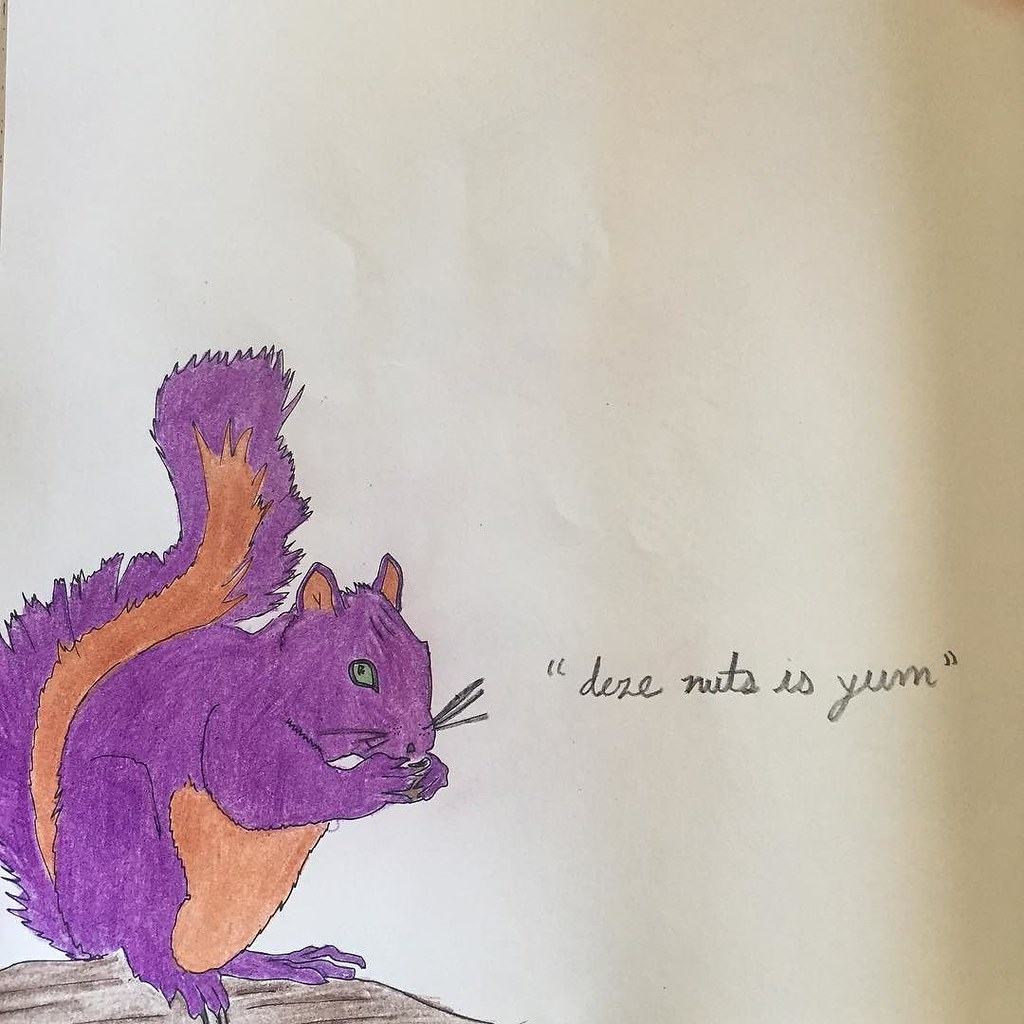This image showcases a colored pencil and pen-and-ink drawing of a whimsical purple squirrel. The squirrel, outlined carefully in pen and ink, stands in the bottom left corner of a white sheet of drawing paper, possibly resembling copy paper. It is perched on a textured rock or wooden surface, holding a nut close to its mouth. The squirrel's body is predominantly colored in purple, while its belly, a stripe along its tail, and the insides of its ears exhibit a light brown hue. Notably, the squirrel has a green eye that gazes directly at the viewer, adding a touch of liveliness to the illustration. To the right of the squirrel, a playfully written caption in cursive says, "D-E-Z-E, nuts is yum," humorously mimicking the popular phrase "deez nuts." The paper's natural white background further accentuates the vibrant colors of the drawing, which might initially give the impression of a coloring book illustration due to its precision and charm.